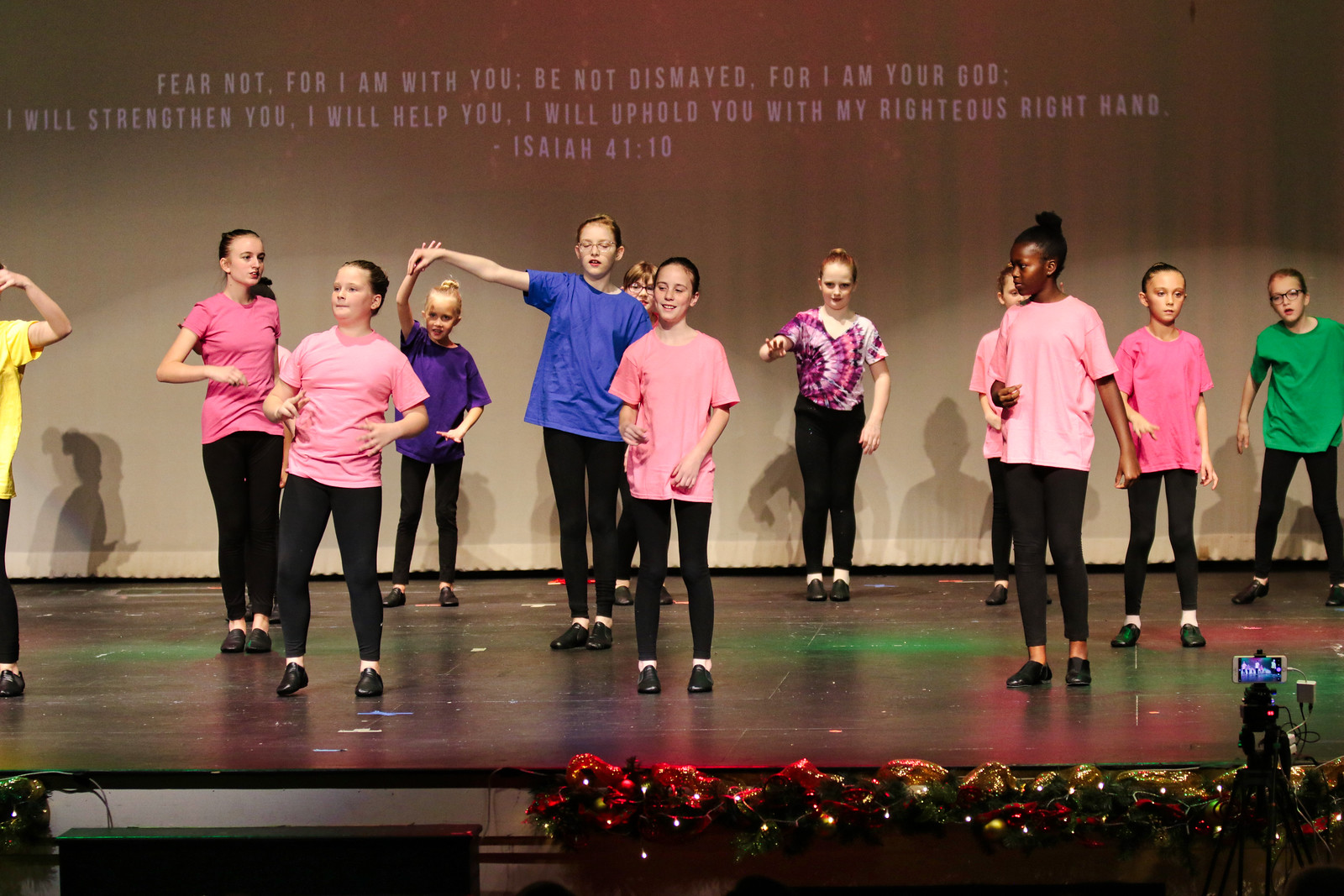This horizontally aligned rectangular image features a group of pre-teen girls, possibly aged 8 to 12, standing on a black, worn-looking stage, engaged in what appears to be a dance performance or practice session. The stage is adorned with festive Christmas decorations, including plants illuminated by little lights and flowers. The girls are dressed in various colored t-shirts that include pink, blue, purple, green, yellow, and tie-dye, paired with black leggings and black ballet or tap shoes. The girl in the center, wearing a blue t-shirt, has her arm raised, while the others stand attentively.

Above them, a Bible verse from Isaiah 41:10 is projected onto a white curtain, which appears pinkish at the top due to overhead lighting. The verse reads, "Fear not, for I am with you; be not dismayed, for I am your God. I will strengthen you, I will help you, I will uphold you with my righteous right hand." The attentive focus of the girls on stage contrasts with the colorful light spots on the stage floor, creating a vibrant yet earnest atmosphere captured by cameras recording the scene.